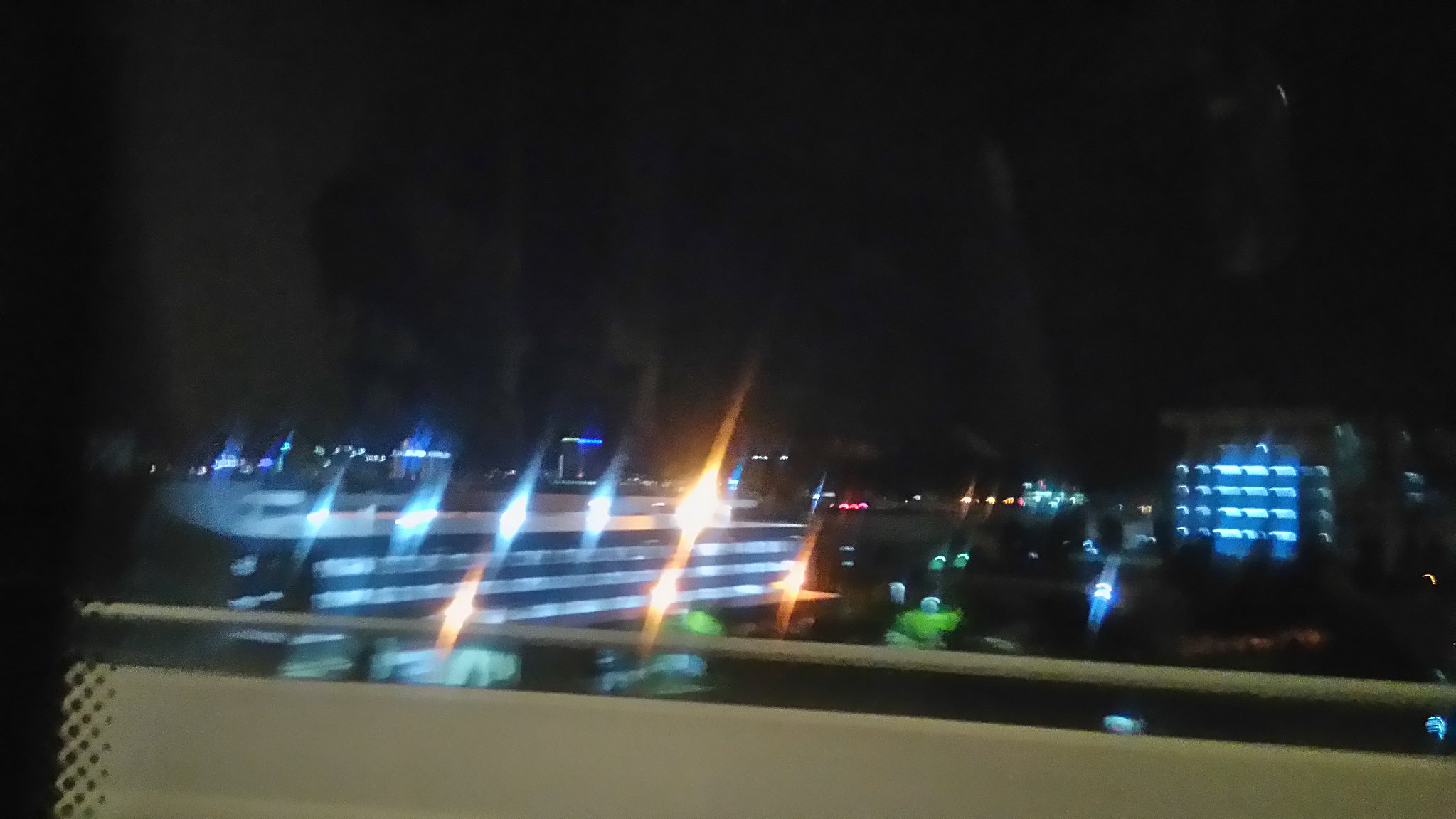A captivating nighttime cityscape is viewed from a high vantage point, likely from a tall building. The perspective reveals the rooftops of several multi-story buildings below. A prominent white rail in the foreground suggests the photo was taken through a window or from a balcony. The city is illuminated with a blend of vibrant lights: numerous blue lights dominate the scene, interspersed with a handful of orange and green lights. The sky is an inky black, enhancing the brilliance of the urban illumination. In the distance, a few skyscrapers pierce the night sky, their tops aglow with white and blue lights. Among them, one building stands out with red lighting, while another features a mix of orange and blue hues, creating a striking contrast in the city's nighttime panorama.